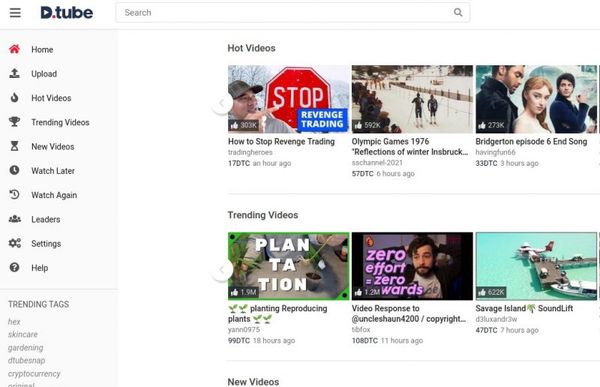In this image, a webpage titled D-Tube is prominently displayed. The D-Tube logo, styled in navy blue, is located in the upper left corner. The overall theme of the website is minimalist, with a predominantly white background. The central portion of the page showcases several video thumbnails, each representing different content.

On the left side of the page, there's a comprehensive navigation menu featuring several sections: Home (currently active), Upload, Hot Videos, Trending Videos, New Videos, Watch Later, Watch Again, Leaders, Settings, and Help. Below this menu, a list of Trending Tags is visible, including topics such as Hex, Skin Care, Gardening, D-Tube Snap, and Cryptocurrency, with additional tags cut off from view.

At the top of the page, there is a search bar available for finding specific videos. The main content area features a section labeled "Hot Videos," displaying three specific videos: "How to Stop Revenge Trading," "Olympic Games 1976," and "Bridgerton Episode 6 End Song." Below this, the "Trending Videos" section lists "Plantation," "Video Response to Uncle Sean 4200," and "Savage Island Sound Lift."

The overall design and layout closely resemble that of YouTube, but with distinct branding as D-Tube, affirmed by the logo in the upper left corner. This suggests that D-Tube operates similarly to YouTube, serving as a platform for video sharing and viewing.